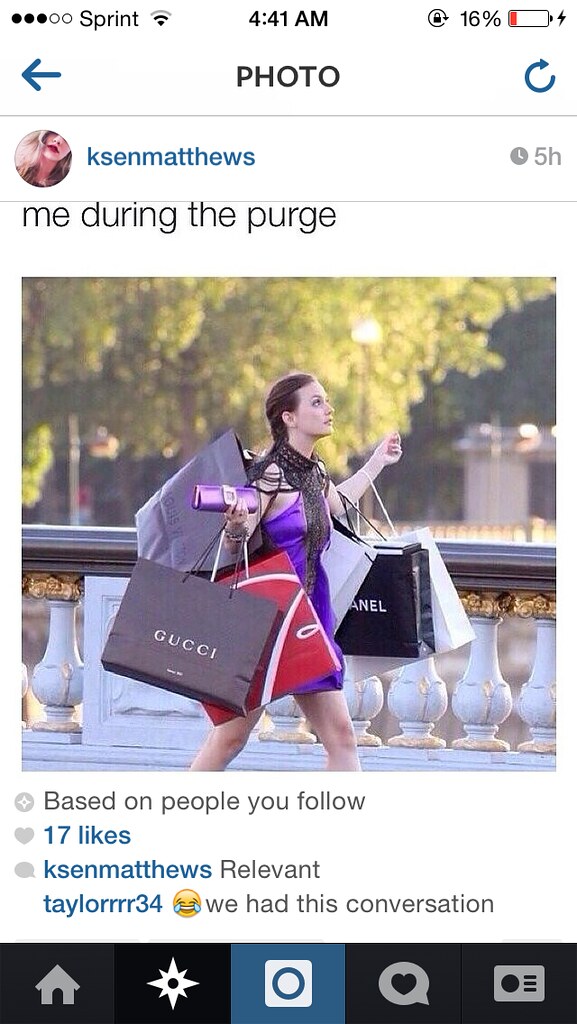The image depicts a screenshot from a social media post taken at 4:41 a.m. on a phone with 16% battery remaining, using the carrier Sprint. The profile picture and name, "KSEN Matthews," are visible in the top left corner. The post features a photograph of a woman with brown hair, wearing a short purple dress with a string top and a brown scarf, walking across a white bridge with green leaves in the background. She is centered in the image, holding six large shopping bags in various colors (brown, red, black, white, and gray) from high-end brands like Chanel and Gucci, along with a stylized purple purse. The caption on the social media post reads, "me during the purge." The interface displays likes, comments, an emoji, and information about followers, suggesting it has 17 likes and that Taylor 34 left a comment saying, "we had this conversation."